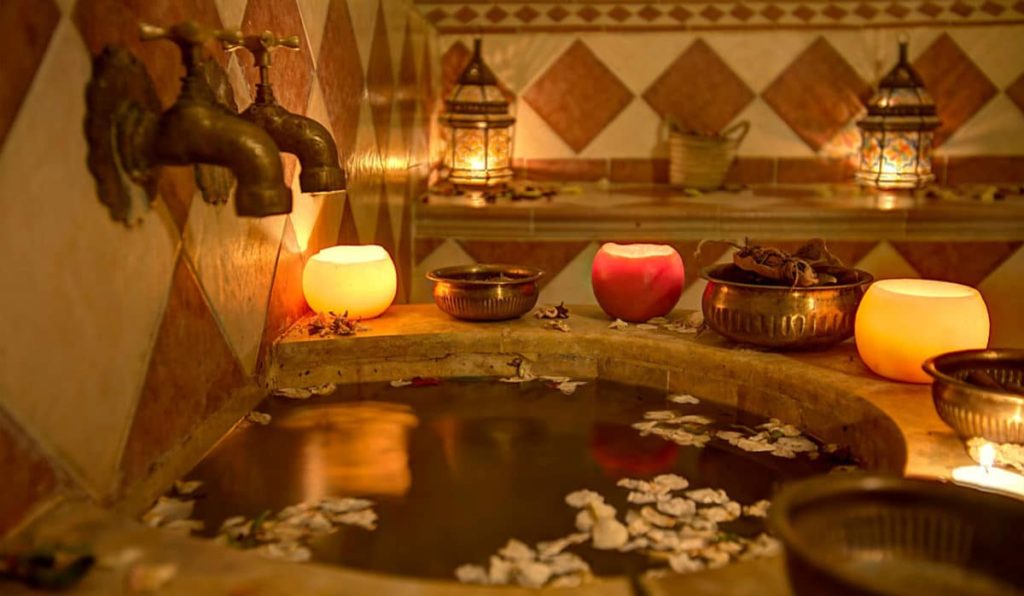The picture depicts a unique and ornately styled bathroom or spa-like setting. The left wall features an intricate design made of diamond-shaped bricks in varying shades of light and dark brown. Affixed to this wall are two vintage-style bronze faucets positioned above a semi-circular sink basin. The basin is filled with a dark liquid, possibly water, on which flower petals and a light brown substance float. Along the edge of the sink, various items are neatly arranged: a circular bowl containing herbs, a lit yellow candle, and a light-up yellow container. A basket brimming with leaves sits near the center of the counter. Additional decor includes a red candle, a yellow candle, and multiple bronze, gold, and silver bowls—some of which contain leaves or other undefined items. Two ornate lanterns adorn a ledge against the far wall, adding to the ambient lighting provided by the multiple candles scattered throughout the space. The overall atmosphere is ambient and relaxing, with a mix of natural and vintage elements meticulously arranged.